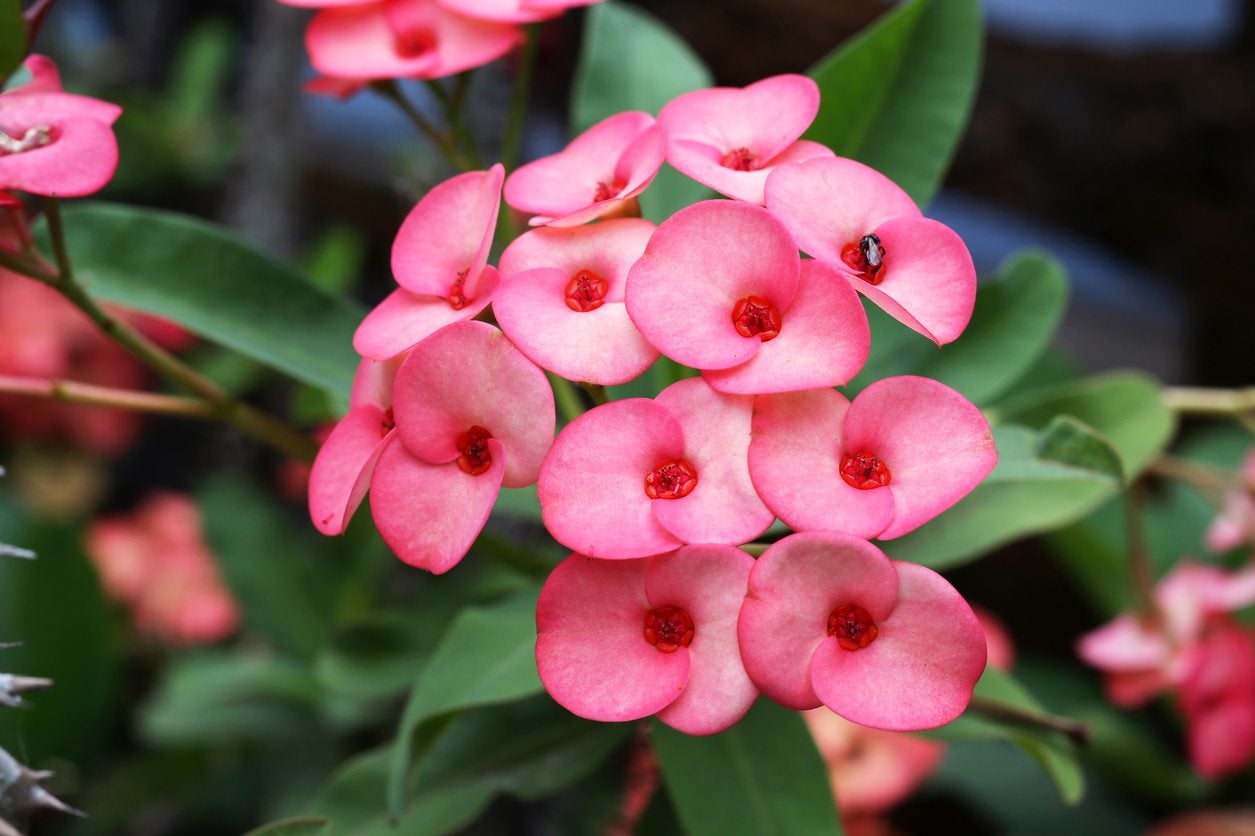This photograph showcases a close-up view of a striking pink plant adorned with clustered flowers. Each flower in the cluster features two petals, which have a gradient from darker pink on the outer edges to lighter pink towards the center. The vibrant red core of the flowers stands out, hinting at where nectar might be found. The main flower cluster, comprising 12 to 14 flowers, dominates the foreground, while additional clusters and green leaves recede into a softly blurred background. The green leaves display a variegated pattern with a central stripe and perpendicular branches. A small bug, possibly a fly, is visible interacting with one of the flowers on the right side of the image, adding a touch of natural interaction. In the bottom left corner, the sharp tips of a spiky plant intrude, adding texture and contrast to the otherwise soft floral scene.